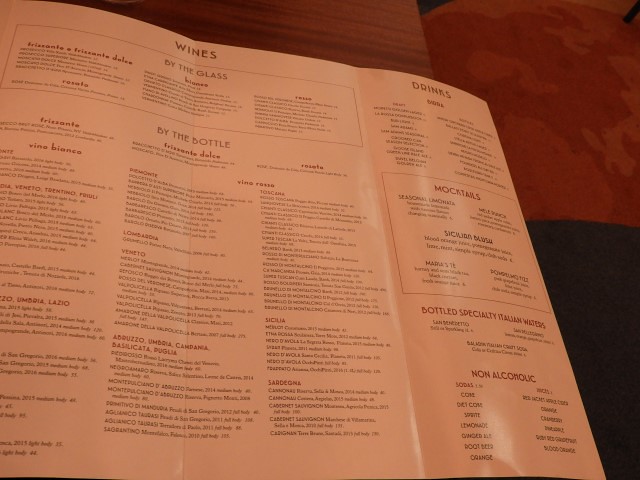This photograph captures an extensive wine and drinks menu from a restaurant, displayed on a single large sheet of paper folded into thirds, much like a letter-sized document. The background reveals hints of a restaurant setting, with a streak of reddish-pink ambient lighting, a glimpse of a table, and a somewhat reddish carpet setting the scene.

The wine section dominates the menu, occupying two-thirds of the document, while the remaining one-third is dedicated to other beverages. The wine list is meticulously organized, featuring categories for wines by the glass and several others by the bottle. Each type of wine listed comes with a subheading, indicating the variety, and includes several selections with their respective prices.

The drinks section, segmented into four main categories, includes options for vodka, mocktails, specialty bottled Italian waters, and non-alcoholic beverages. Each category offers a curated selection of drinks, catering to diverse tastes and preferences. This detailed menu not only showcases a broad selection of wines and beverages but also hints at a sophisticated dining experience.